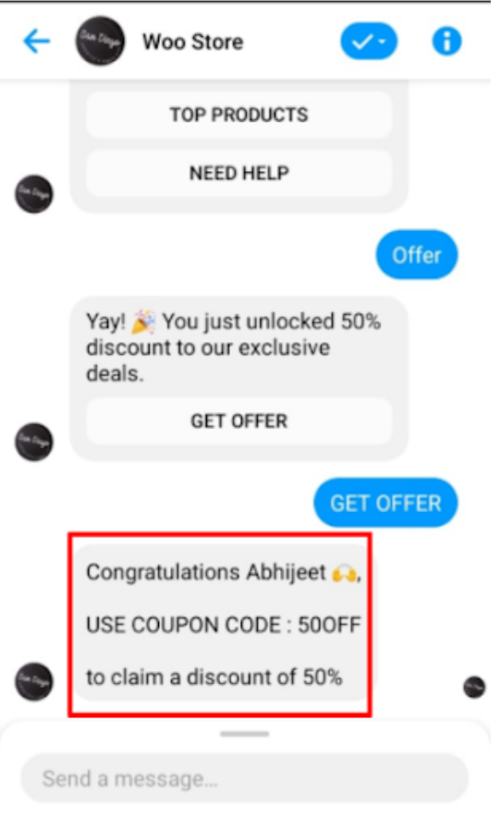The image displays a text message with a distinct interface. At the top, there's a horizontal black line stretching from left to right, overlaying a white background. A blue arrow pointing left is situated beside a black circle, adjacent to the text "The Wool Store." Below, there's a blue box with a checkmark, followed by another blue box containing a lowercase "i."

Further down, the screen shows a text message originating from "The Wool Store," highlighting their top product and a call to action for assistance with a blue text box labeled "Offer." Subsequently, in a gray-colored text box, the message reads: "Yay, you just unlocked a 50% discount to our exclusive deals," accompanied by a blue button labeled "GET OFFER" in capital letters.

In another gray text box underneath, the message continues with: "Congratulations, your coupon code is $5.50 off to claim a discount of 50%." At the bottom, there is a text box prompting the user to "Send a message."